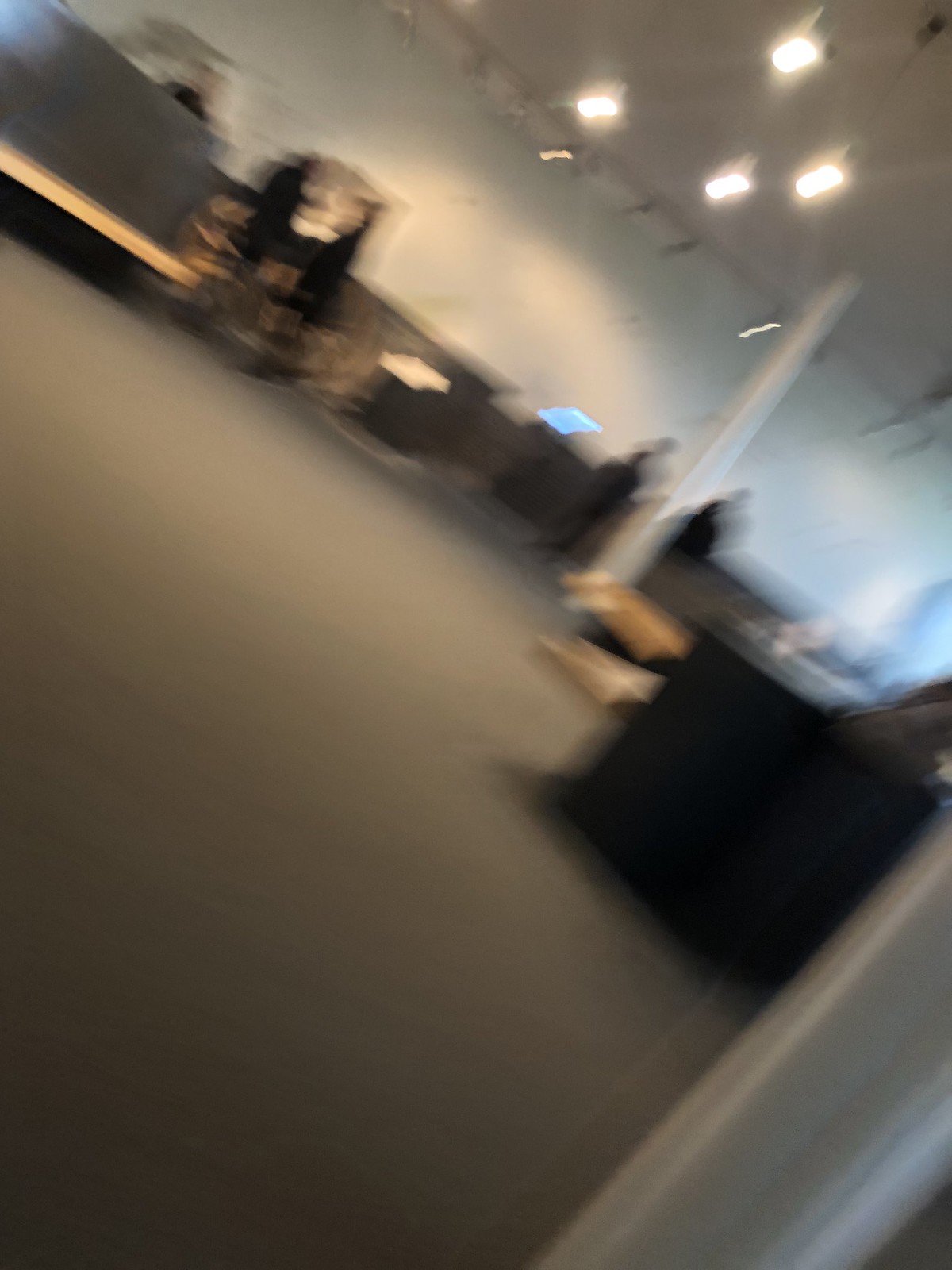This is a very blurry photograph of a large indoor area that resembles a warehouse or possibly a theater backstage. The flooring is gray, though the strong blur obscures its exact material. The space feels cavernous, with light-colored walls and ceiling. Overhead, to the top right, there are hanging spotlights, likely meant for a show, casting light across the room. To the right side of the image, a black countertop or desk can be seen, while a small section of a white doorframe is visible towards the bottom right, where it appears to be dusted with black particles. Various light-colored beams or poles are scattered around the area. In the center, more toward the top, there's a light blue square that looks like a screen. There are also several people in the image, appearing as blurred dark figures. The photograph seems to have been taken at an angle, possibly from someone who had just entered through the doorway, giving the image a sense of secrecy or hurried movement.